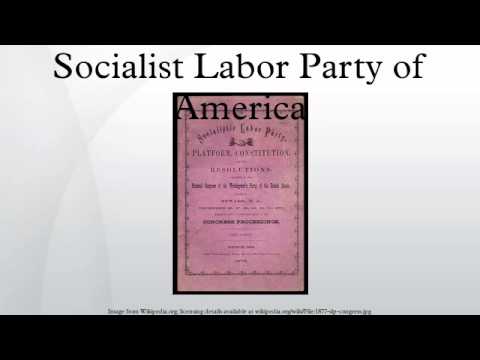This rectangular image features a document presentation with a thin black bar at both the top and bottom, set against a light gray background with a gradient and some geometric curves. Centrally positioned at the top, clear black text reads "Socialist Labor Party of America." Below this, there is a scan or picture of a historical document, possibly a pamphlet, attributed to the Socialist Labor Party of America. The document is pinkish in hue, designed with a professional, serif font that resembles Times New Roman. The print on the document appears to be created using a traditional printing press, though it is too small to read the specific details. At the bottom, there is another line of text, also too tiny to decipher. The entire layout gives the appearance of a PowerPoint slide or a screenshot from a video, emphasizing the document's historical and cultural significance.